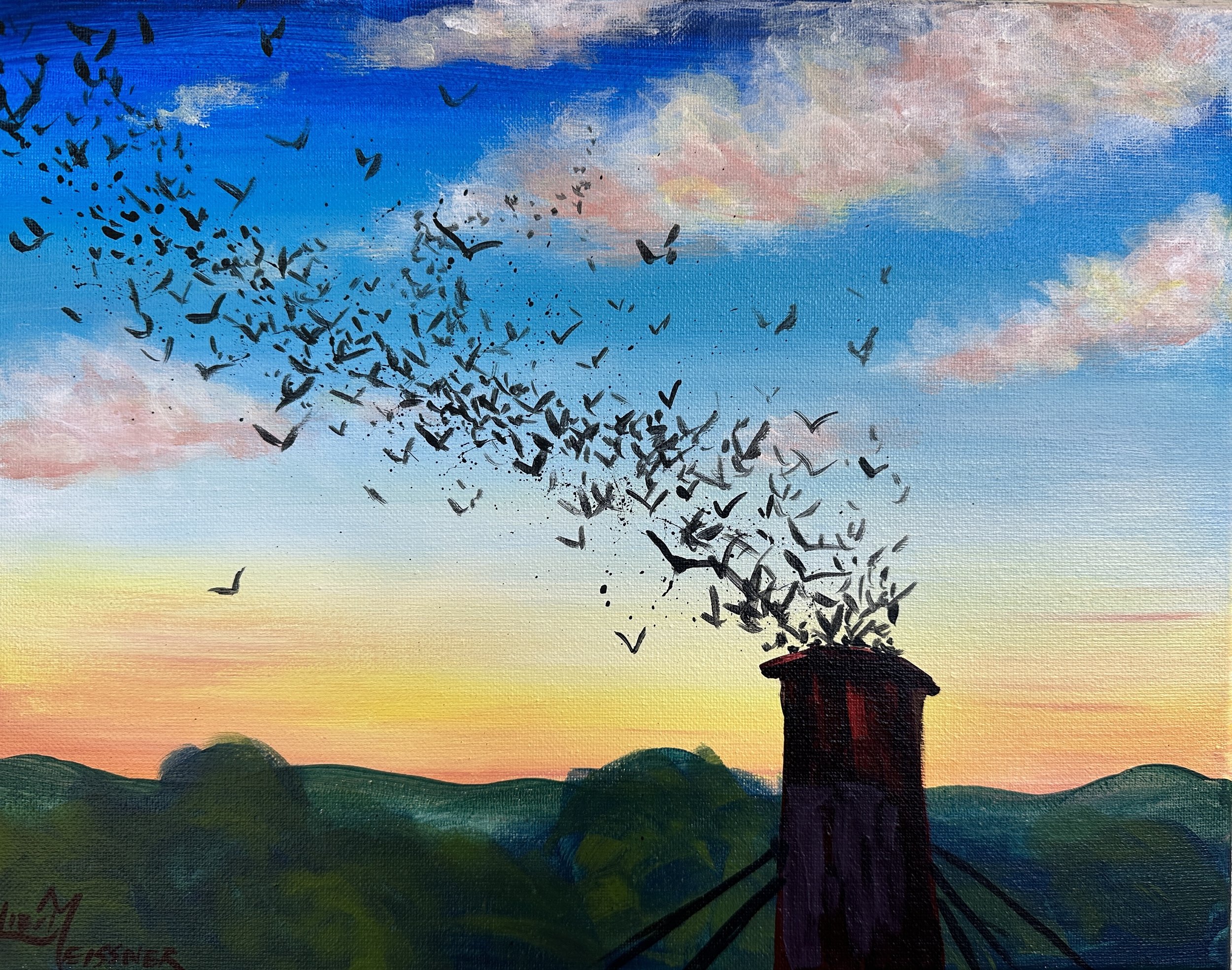This painting depicts a dramatic landscape dominated by a tall, red structure resembling a chimney or possibly a forestry watchtower, positioned in the lower right corner. The sky features a striking gradient transitioning from deep, royal blue at the top, dotted with white clouds, to warm, sunset hues of orange and yellow nearer to the horizon. Below this vibrant sky, a series of rolling hills or mountains, painted in dark green and blue tones, stretch across the lower part of the image. A large flock of black birds is seen emerging en masse from the red structure, soaring upwards and towards the top left corner of the painting, creating a dynamic sense of movement against the tranquil backdrop.